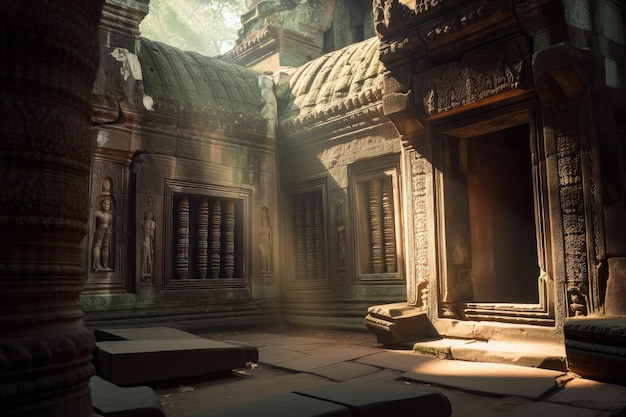The image depicts a CGI-rendered or digitally-created ancient stone temple combining elements of Egyptian and Roman architectural styles. The structure boasts intricate chiseling and artwork with detailed carvings in a relief style adorning its walls. The building features curved rooflines, visible in two tiers, and statues placed between framed pillars. The color palette consists of various shades of gray, brown, tan, and dark brown, contributing to its weathered, old appearance. The ground comprises large, flat, rectangular stone pieces that are uneven in places. On the right side of the image, an open doorway with decorative trim invites the viewer's gaze, while a sliver of blue sky with clouds and a hint of a green tree peeks through near the top left. Sunlight streams through this gap, casting rays onto the front stone step, enhancing the temple's ancient and mystical aura.